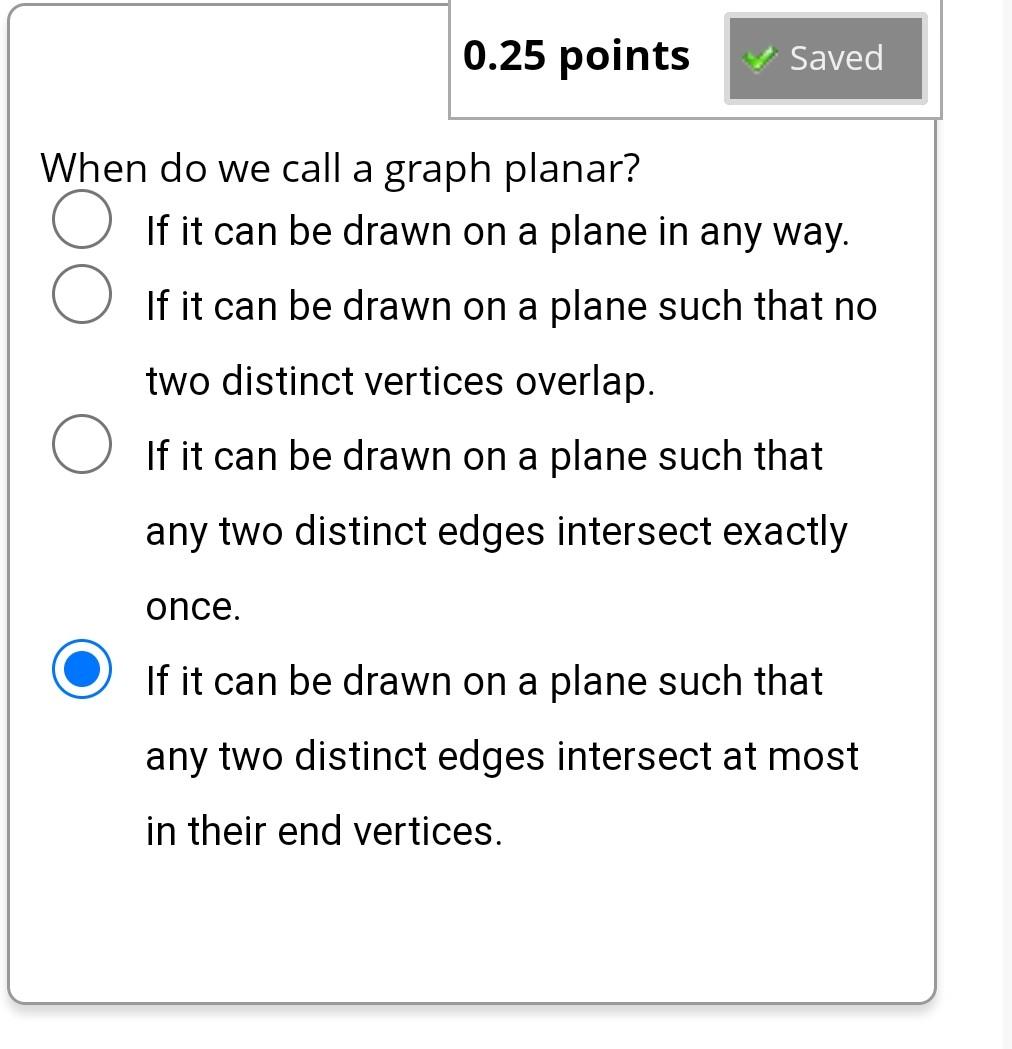The image features a detailed diagram with multiple sections and annotations, set against a white background. 

At the top of the image, there is a square with a gray border, though its top-right corner is partially cut off. This gives way to a small section that is bordered off from the rest of the diagram. Within this section, "0.25 POINTS" is written in dark, bold black letters.

Next to this section is a silver-bordered rectangle with a dark gray or dark silver background. Inside this rectangle, there is a green check mark on the left, and the word "Saved" in white with a capital 'S' to the right of the check mark.

Below this segmented area, occupying the main part of the image, is a larger white background square. At the top of this main section, it reads "When do we call a graph planar?" in capital letters.

Adjacent to the left of this main text, there is a gray-bordered circle with a white interior. Next to this circle, the text reads, "If it can be drawn on a plane in any way." The sentence starts with a capital 'I.'

Below this are two more similarly styled gray-bordered circles with white interiors, each accompanied by descriptive text. The first of these circles states, "If it can be drawn on a plane such that no two distinct verticals overlap," again starting with a capital 'I.' The second circle says, "If it can be drawn on a plane such that any two distinct edges intersect exactly once," also beginning with a capital 'I.'

Additionally, there is a final circle that stands out with a blue border. Inside this circle, there is a small, dark blue solid circle, and in between the dark blue circle and the light blue border, there is a white space. Next to this blue-bordered circle, the text reads, "If it can be drawn on a plane such that any two distinct edges intersect at most in their end vertices." Note that "vertices" was misspelled as "verdicts" in the original caption.

Overall, the image is a detailed exploration of the conditions under which a graph can be considered planar, presented through a series of textual and graphical elements.